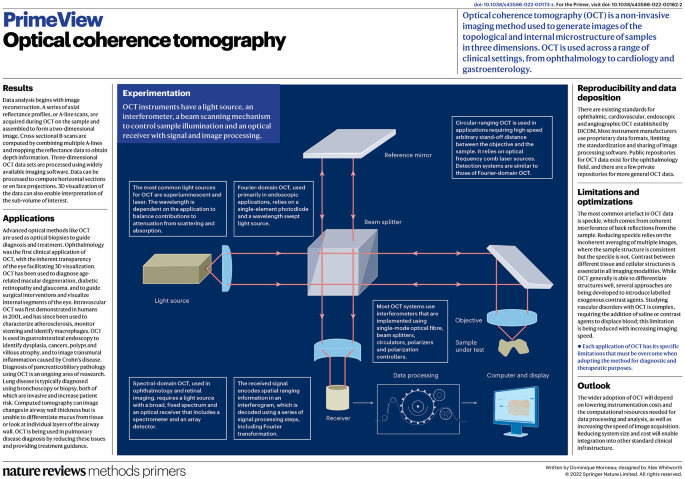The image portrays a detailed page from a textbook or scientific journal, showcasing an article on Optical Coherence Tomography (OCT). At the top, "Prime View" is prominently displayed in blue text, followed by the title "Optical Coherence Tomography" in black. The article explains that OCT is a non-invasive imaging method used to generate detailed three-dimensional images of topological and internal microstructures, with applications spanning ophthalmology, cardiology, and gastroenterology.

Centrally featured is a comprehensive diagram on a dark blue background, illustrating the components of an OCT instrument. The diagram includes a white cube at the center, a light source on the left side, and multiple coral-colored lines with arrows indicating the light paths. To the right, a white plate and a round blue lens are depicted. Surrounding this diagram are numerous labels and paragraphs detailing various aspects of OCT. 

On the left side of the page, the headings "Results" and "Applications" introduce their respective sections. On the right side, the headings "Reproducibility and Data Deposition," "Limitations and Optimizations," and "Outlook" are listed, each accompanied by explanatory text. At the very bottom of the page, "Nature Reviews" is printed in black text, with "Methods Primers" in standard typeface. Overall, the image provides an in-depth look at both the theoretical and practical elements of OCT technology.